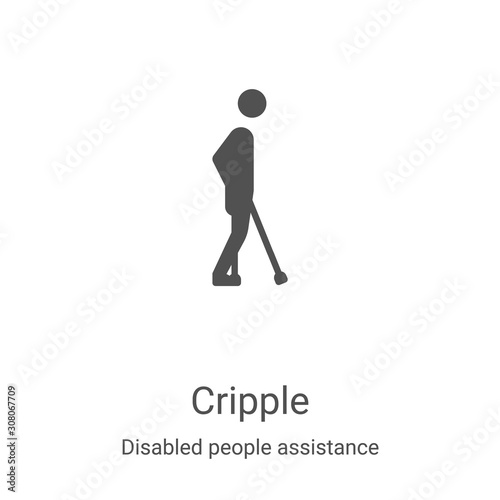This image is a simple black and white illustration designed to represent "crippled disabled people assistance." The icon depicts a stylized figure of a person with a detached circular head, walking with a cane, symbolizing the need for assistance in mobility. The body and legs are rendered in dark gray, while the background remains white. Below the figure, the words "cripple disabled people assistance" are written, with "cripple" in larger text and "disabled people assistance" in smaller letters underneath. A barely visible watermark, featuring indistinguishable letters like "E" and "S," runs across the image at a 45-degree angle. Vertically aligned in small text on the bottom left corner, it reads "Adobe Stock 308067709." This icon resembles the sort of generic symbols often used for public signs, suggesting it might be a new symbol representing disabled individuals needing assistance.